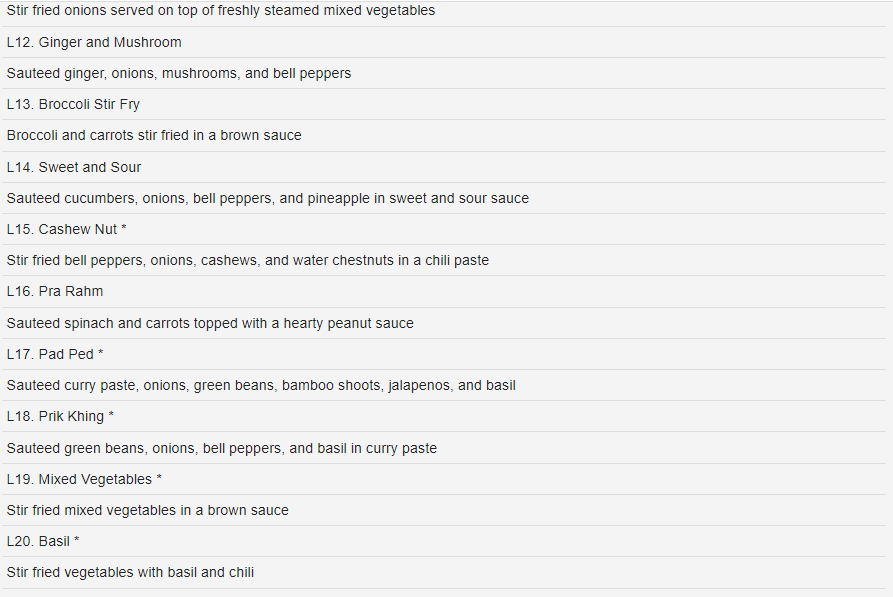Here is a detailed, cleaned-up descriptive caption for the voice-given image of the menu:

---

**Image Caption: Detailed Restaurant Menu Listing Various Stir-Fried Dishes**

The image shows a comprehensive menu, seemingly from a restaurant, featuring an array of stir-fried dishes, each designated by a unique identifier (e.g., L12, L13, etc.). The menu items are divided with lines in between each entry, and the dishes include a variety of fresh ingredients and flavorful sauces. Below is a detailed description of each item listed:

- **L12 - Stir-Fried Onions**: This dish consists of stir-fried onions served atop a medley of freshly steamed vegetables, offering a simple yet satisfying combination.
  
- **L13 - Ginger Mushrooms**: Sauteed with ginger, onions, mushrooms, and bell peppers, this dish provides a savory blend of aromatic and umami flavors, perfect for mushroom lovers.
  
- **L14 - Broccoli**: Featuring stir-fried broccoli and carrots cooked in a rich brown sauce, this item brings a nutritious and flavorful option to the table.
  
- **L15 - Sweet and Sour**: A delightful mix of sauteed cucumbers, onions, bell peppers, and pineapple, all enveloped in a tangy sweet and sour sauce.
  
- **L16 - Cashew Nut**: This dish integrates stir-fried bell peppers, onions, cashews, and water chestnuts, all seasoned with a spicy chili paste for an added kick.
  
- **L17 - Para Ham**: Comprising sauteed spinach and carrots, this dish is enriched with a hearty peanut sauce, providing a rich and creamy taste.
  
- **L18 - Pet Pad Pet**: Sautéed curry paste enhances the flavors of onions, green beans, bamboo shoots, jalapenos, and basil, creating a vibrant and spicy dish.
  
- **L19 - Prick King**: Featuring sautéed green beans, onions, bell peppers, and basil, this dish is cooked in a savory curry paste, offering a burst of rich spices and textures.
  
- **L20 - Mixed Vegetables**: A simple yet appetizing combination of stir-fried mixed vegetables prepared in a brown sauce, ideal for a nutritious and balanced meal.
  
- **L21 - Basil**: Stir-fried vegetables combined with basil and chili, delivering a fragrant and mildly spicy profile.

The detailed descriptions emphasize the variety and richness of flavors and ingredients highlighted in this restaurant menu. Each dish offers a unique taste experience, catering to a range of palates.

---